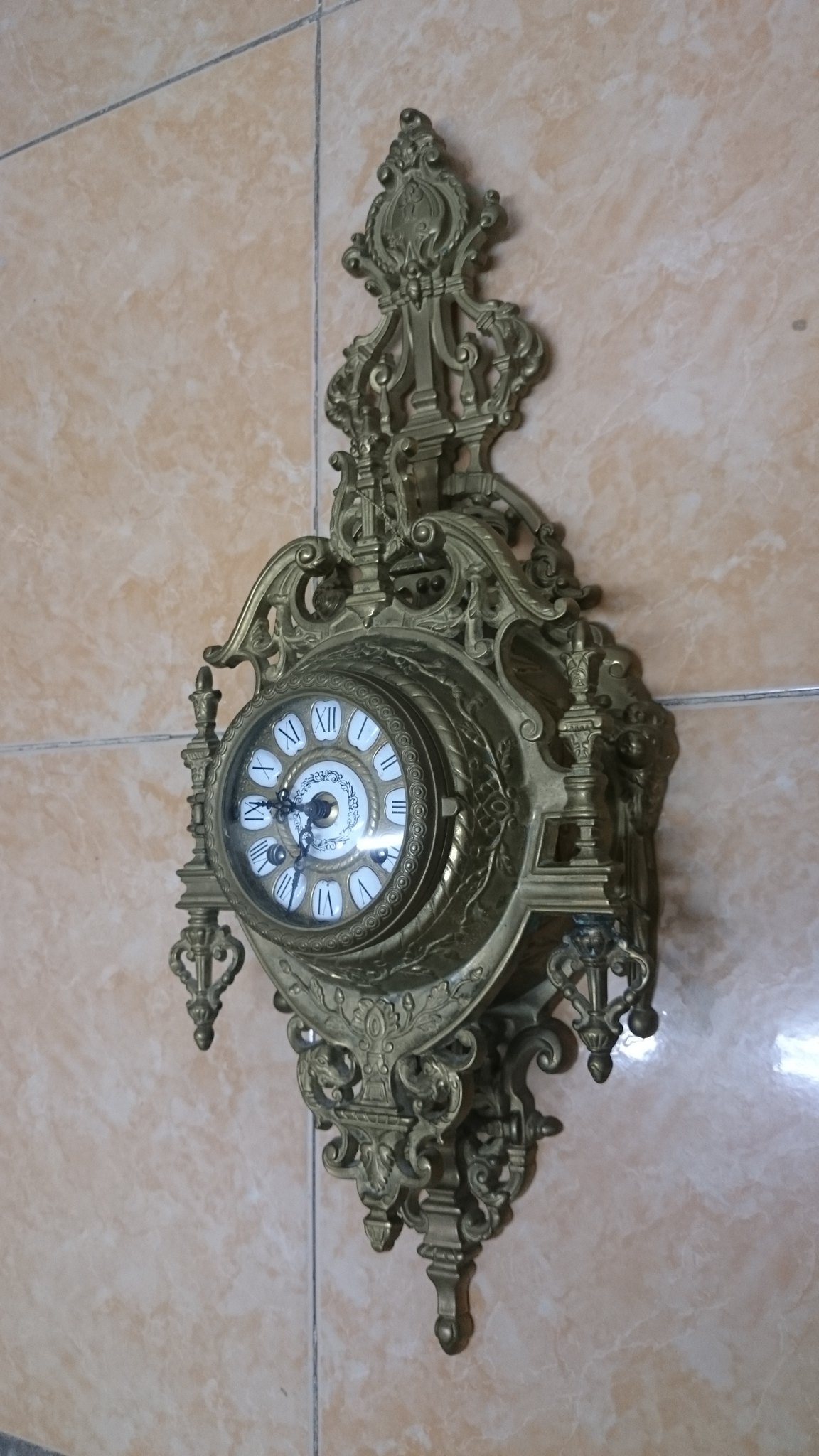In this detailed image, we observe an antique-style clock prominently displayed against a background patterned with light brown and white streaked square tiles. The clock's frame features intricate line designs and is finished in a rich brown color, contributing to its vintage appeal. At the center of the clock, Roman numerals replace the traditional numbers, each highlighted within its own white square, creating a striking contrast against the clock face. The clock's black hour hand points to where the nine would be, while the black minute hand indicates the seven, adding to the timeless elegance and charm of the piece.